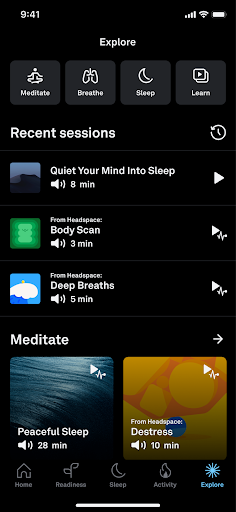This image is a vertical screenshot of a mobile phone interface with a jet black background. The time displayed at the upper left-hand corner is 9:41, and at the top right-hand corner, there are three icons including a battery icon. Centrally positioned, the title of the page reads "Explore."

Below the title, there are four dark gray buttons each with corresponding icons labeled as Meditate, Breathe, Sleep, and Learn. Directly beneath these buttons, the text "Recent Sessions" appears in large, bold white font. Adjacent to this text on the right side, there is an icon featuring a circle with an arrow encircling a time symbol.

The section following "Recent Sessions" lists three playable tracks. Each track has a thumbnail image to its left. The track titles are:
1. "Quiet Your Mind Into Sleep" with a displayed duration.
2. "Body Scan" with its time duration indicated.
3. "Deep Breaths," also showing its duration. Each track listing ends with a right-facing arrow.

Further down, there is a section labeled "Meditate." This section contains two large square icons representing sound recordings. The left square is labeled "Peaceful Sleep" with a recording length of 28 minutes, while the right square is labeled "De-Stress" with a 10-minute duration.

At the bottom of the page, a navigation bar displays five icons with text labels: Home, Readiness, Sleep, Activity, and Explore. The Explore icon is highlighted in light blue and features a sun logo, indicating the current active category. A thin, horizontal white line runs across the lower center of the image.